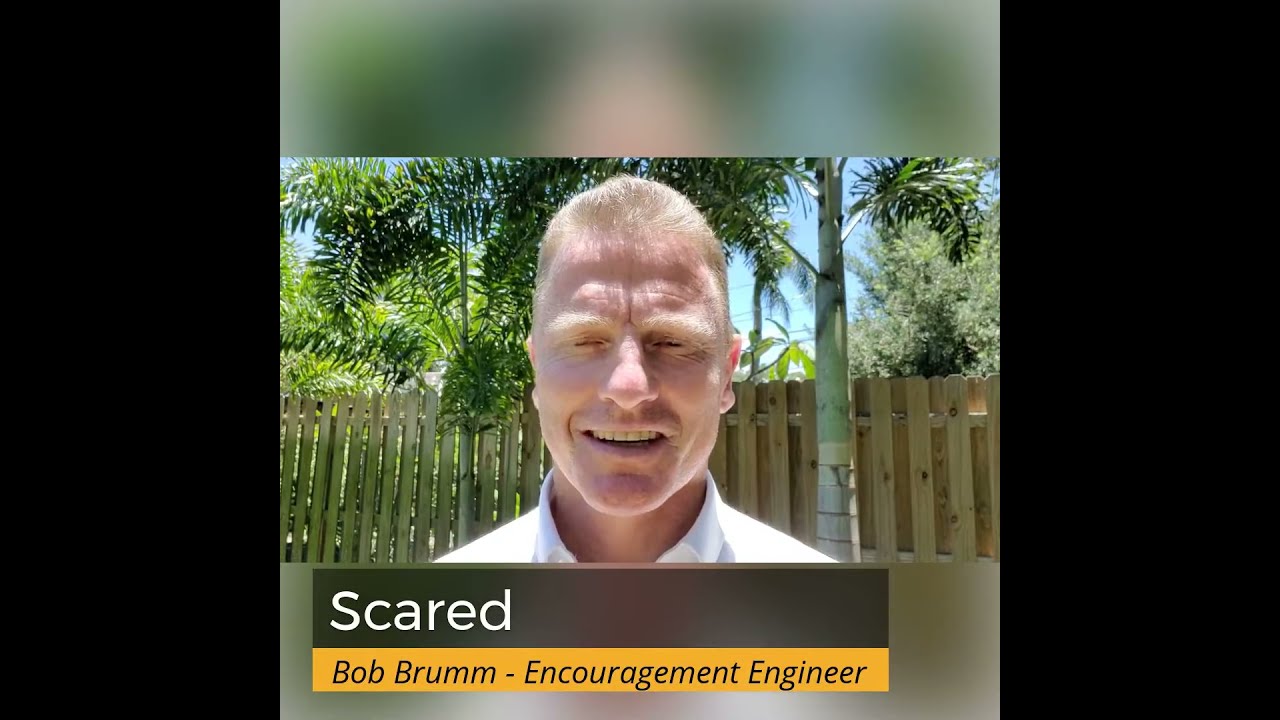The photograph depicts a Caucasian man with very blonde hair and matching blonde eyebrows, captured during the daytime, possibly in a tropical or backyard setting. He is wearing a white dress shirt, and only his head and neck are visible in the image. His eyes are closed, his face is lit from above by sunlight, and he has his mouth slightly open, displaying an ambiguous expression that is neither a smile nor a frown. The background features a wooden fence, green foliage, and trees against a clear, sunny blue sky. The image is framed with large black bars on the left and right sides. Directly below the man is a banner; the top section of the banner is black with the word "scared" written in white letters, and the bottom section is yellow with "Bob Brum, encouragement engineer" written in black letters.